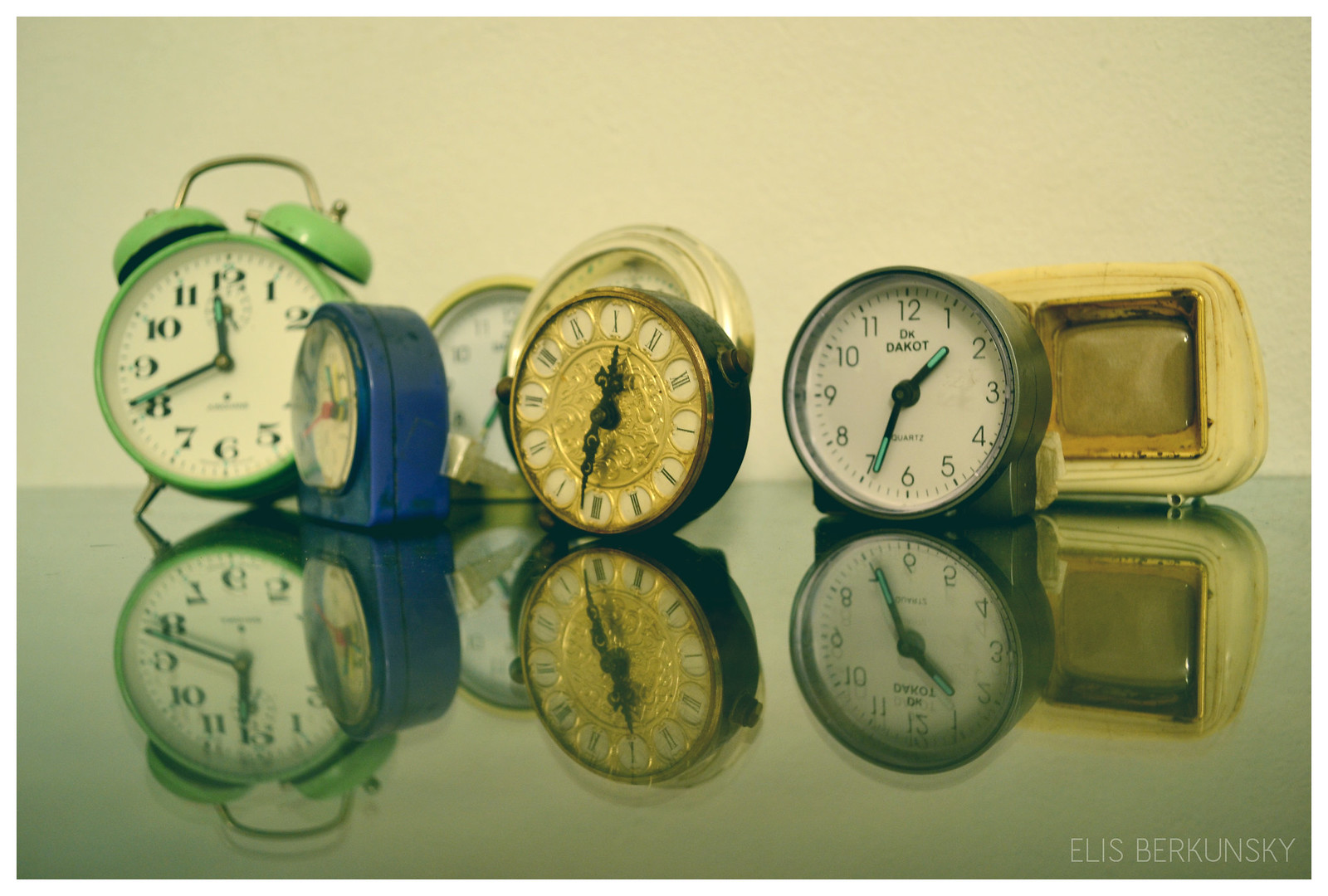This photograph captures an array of vintage-style clocks meticulously arranged on a highly reflective hard surface, where each clock's image is mirrored below it. The backdrop is a subtle, light tan or cream-colored wall, adding a soft warmth to the overall scene.

From left to right, the first clock is a charming, light green vintage alarm clock with a white face and bold black numerals. Its design is accented by two small green alarm bells perched at the 1 o'clock and 11 o'clock positions on top. Moving rightward, we encounter a blue clock angled away from the camera, revealing only its light-colored face partially. Behind it, a light yellow-rimmed clock with a white face peeks through.

Dominating the center is a metallic clock whose face remains hidden by an overlapping gold-faced clock in front of it. This front clock features black Roman numerals encircled by a black rim. To its right, a clock with a white face and black numbers set against a dark gray or black body stands prominently. Lastly, in the background, a square object of a light cream color appears, though its clock face is not visible.

Together, these contrasting clocks create a visually intriguing tableau, each piece adding to the timeless essence of the photograph.